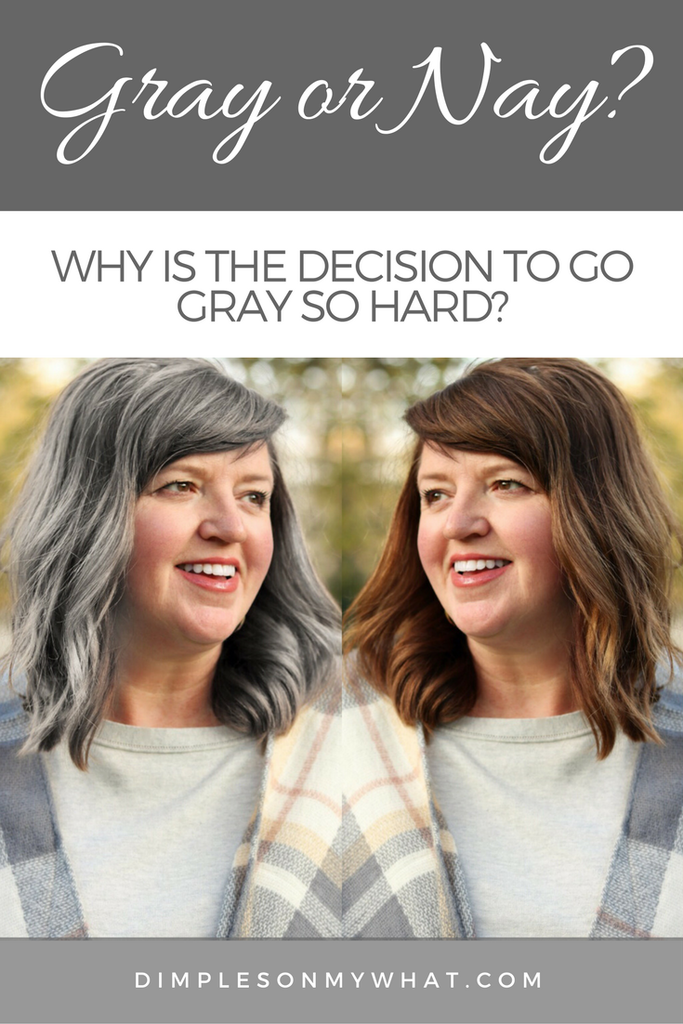The image is an advertisement from dimplesonmywhat.com centered on the theme of deciding whether or not to embrace gray hair. At the top, the ad features a large gray horizontal strip with the white cursive text "Gray or Nay?" Immediately below this, in a thin white strip with gray text, it asks, "Why is the decision to go gray so hard?" The main attraction is a mirror image of the same Caucasian woman, placed side-by-side. On the left, she has gray hair with dark streaks, and on the right, she has light brown hair. Her eyes are brown, her lips are very pink, and she is dressed in a light gray and white plaid jacket over a gray shirt. The woman is set against a daylight background. At the very bottom of the ad, another gray strip with white text displays the URL: dimplesonmywhat.com. The ad seems interactive, encouraging viewers to contemplate or participate in the conversation about going gray.